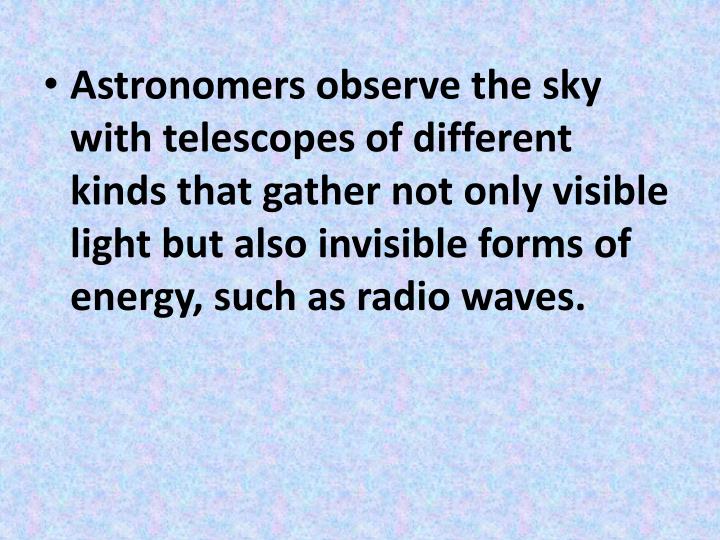The image depicts a rectangular page that appears to be generated from a computer. The background features a subtle, textured mix of light blue, purple, pink, and white, though predominantly bluish in hue. At the top left of the page, there is a black bullet point followed by black text spread over five lines. The text reads: "Astronomers observe the sky with telescopes of different kinds that gather not only visible light but also invisible forms of energy, such as radio waves." The design is simple with no additional images, references, or websites, and the text is aligned to the left. The background, reminiscent of a hazy blue sky, adds a gentle aesthetic contrast to the bold text. The entire image is slightly wider than it is tall.